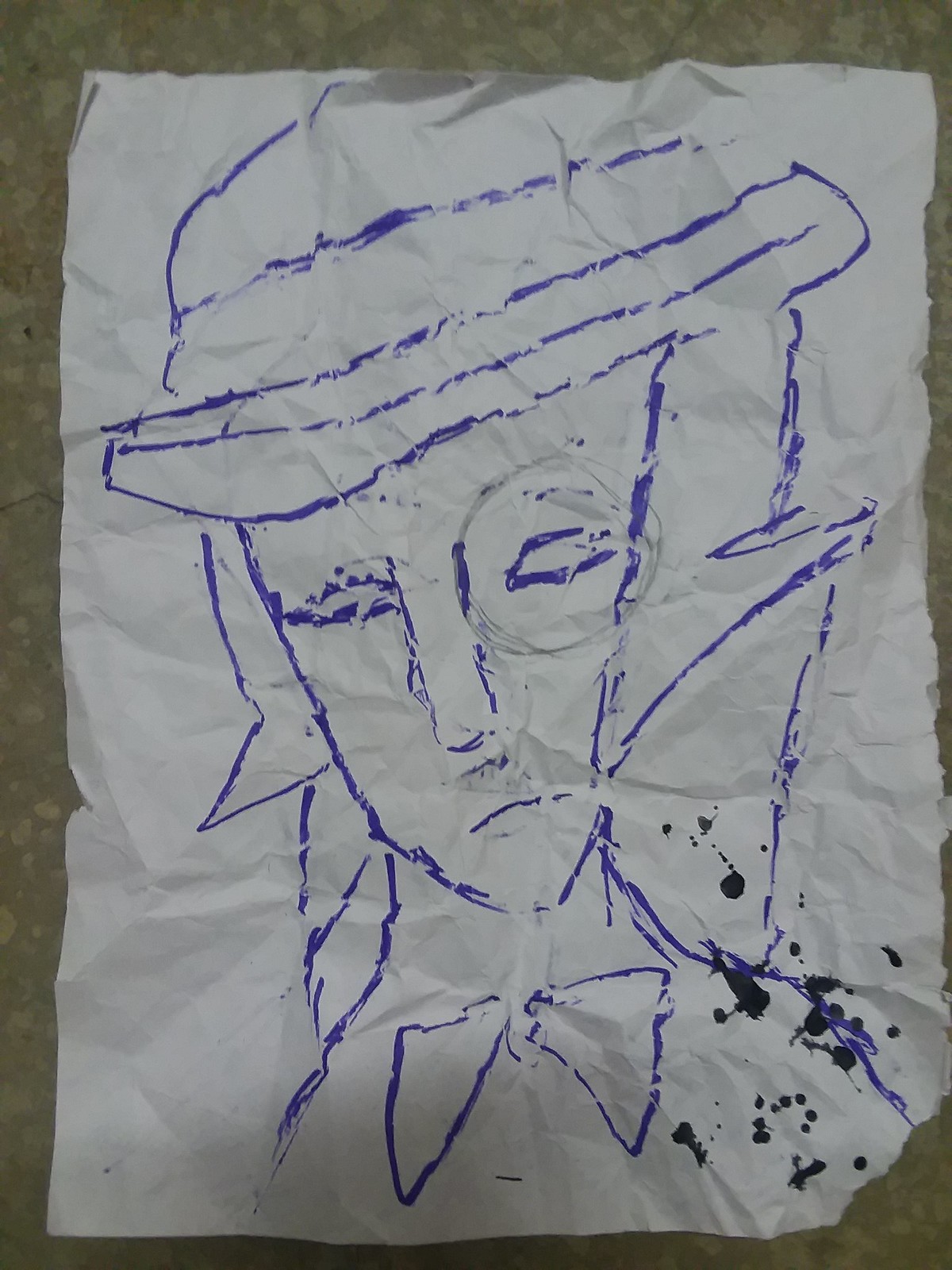This is a photograph of a rudimentary sketch drawn in blue marker on a crumpled and slightly torn white piece of paper. The sketch depicts a person's face, featuring closed eyes, a nose, a mouth, a hat, and a bow tie. The paper shows signs of distress with numerous crinkles and wrinkles, and the edges appear roughly torn, with the bottom right corner significantly damaged. Additionally, there is a noticeable black ink splatter on the bottom right side of the paper. The background of the photograph appears to be a granite countertop, displaying a mixture of off-whites, tans, and darker specks. The drawing, despite its simplicity, clearly portrays the face of a person with distinctive spiky hair on the side of the head.